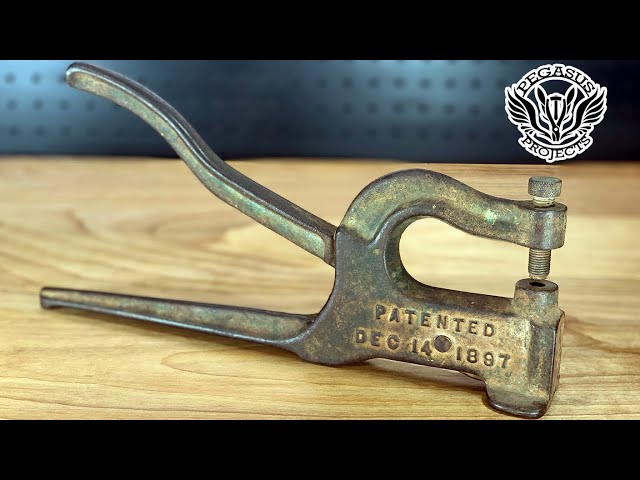This image captures a detailed close-up of an aged, rusted tool resembling a hole punch or an old-fashioned wrench, resting atop a wooden workbench. The metal tool, significantly worn with black and green splotches, boasts a handle reminiscent of a can opener and features an engraved patent date of December 14, 1897. At the top, a screw threads through one hole, with another hole positioned at the bottom, indicating its clamp-like function. The backdrop consists of a dark, pitted wall, creating a rugged contrast. In the top right corner, a logo appears, depicting a forward-facing Pegasus with a bridle and wings extending from its shoulders, encircled by the white text "Pegasus Projects." The photograph is framed by wide black banners at the top and a slightly narrower one at the bottom.